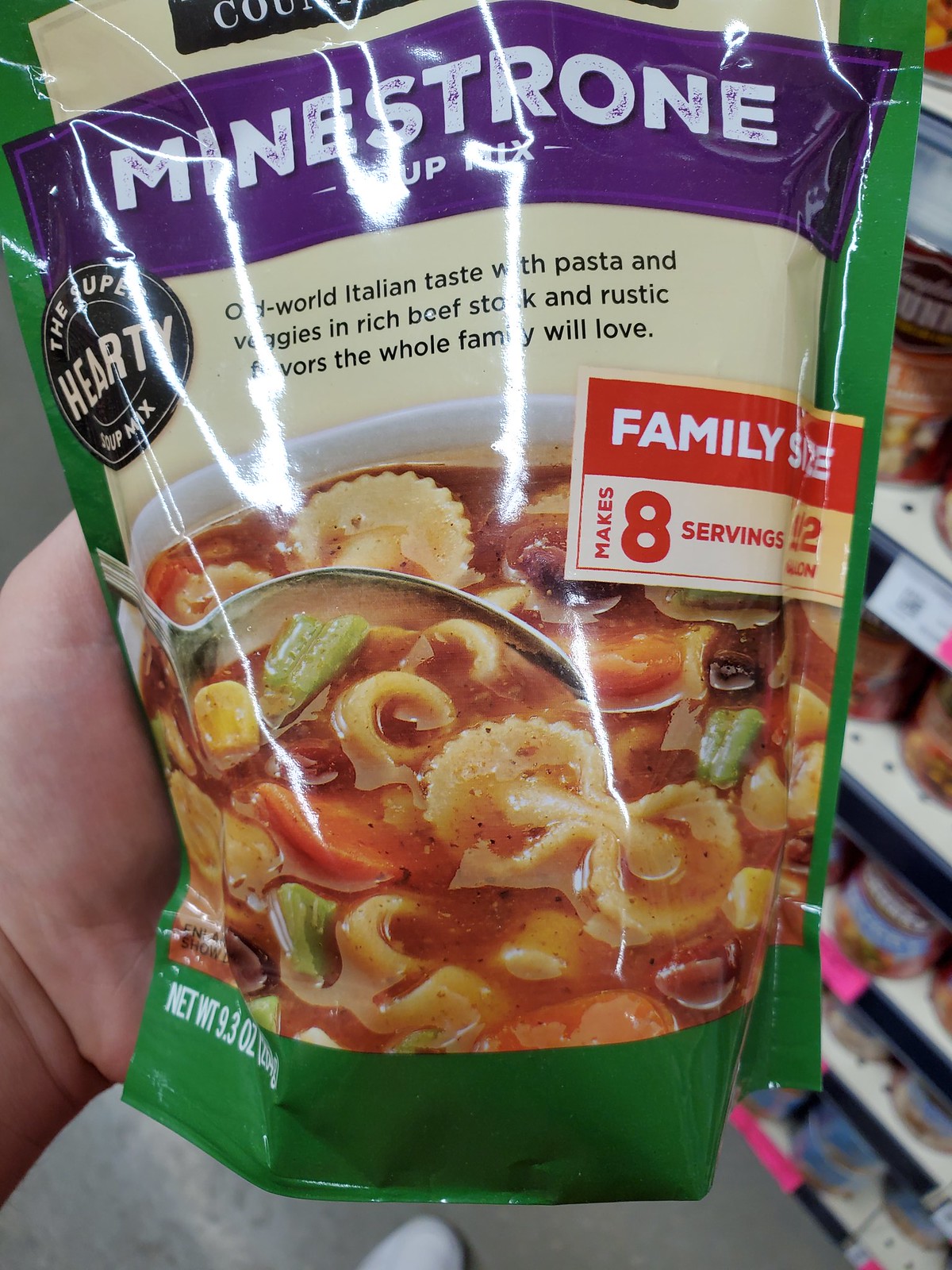In this photograph, a left hand is holding a bag of minestrone soup mix in what appears to be a store aisle with shelves stocked full of various canned soups in the background. The bag prominently features a broad purple stripe near the top with the product name, but the manufacturer's name is obscured. The bag has green edges and a cream-colored central background that reads "Old World Italian taste with pasta and veggies and rich beef stock and rustic flavors the whole family will love." Below, there's a black circle with white text inside that states "The Super Hearty Soup Mix," along with a partial white circle. A picture of the prepared soup in a white bowl is displayed on the front of the bag. There’s an orangey-yellow tab featuring a red rectangle labeled "Family Size," and an outlined red rectangle indicating "Makes Eight Servings." Some additional text is visible but crinkled, making it unreadable. The bag weighs 9.3 ounces. The bottom of the photo includes the photographer’s foot, partially visible on a gray floor.